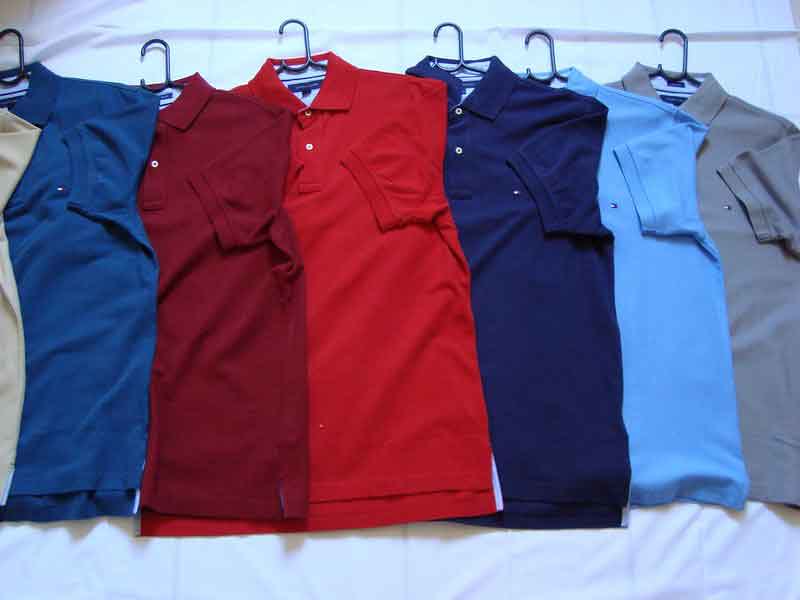In this color photograph, we see a meticulously arranged row of men's polo shirts, all hanging on blue wire hangers, laid out on an off-white, creased fabric that appears to be a bedspread or sheet. The shirts are all short-sleeved and feature small buttons at the collar. From left to right, there is the edge of a tan/beige shirt barely in view, followed by a medium blue shirt. Then, a maroon polo shirt is next to a bright red one. Following the red polo, there is a navy blue shirt, and next to it is a light blue shirt with a small, rectangular emblem on the front. Finally, on the far right, there is a gray, slate-colored polo shirt, also sporting a similar emblem. All the shirts look new and very clean, with their sleeves neatly folded over to touch the chest.